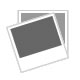In a close-up, vertical image, a person is holding a long, cylindrical object in their left hand, with the thumb propping it up and the fingers wrapping behind it. The object is an antique or artifact characterized by a deep brown-bronze color adorned with intricate ornamental designs. These designs resemble wispy, leaf-like swirls reminiscent of latte art, interspersed with lighter-colored, pearl-like dots. The object narrows slightly as it rises before expanding into a larger, raised ring at its top, which is cut off in the image and exhibits an orangey-bronze hue. The top part reflects light, adding a shiny dimension. This artifact is resting on an off-white surface, with the background featuring a blue wall and a white baseboard to the right, and a vertical white structure in the corner on the left.